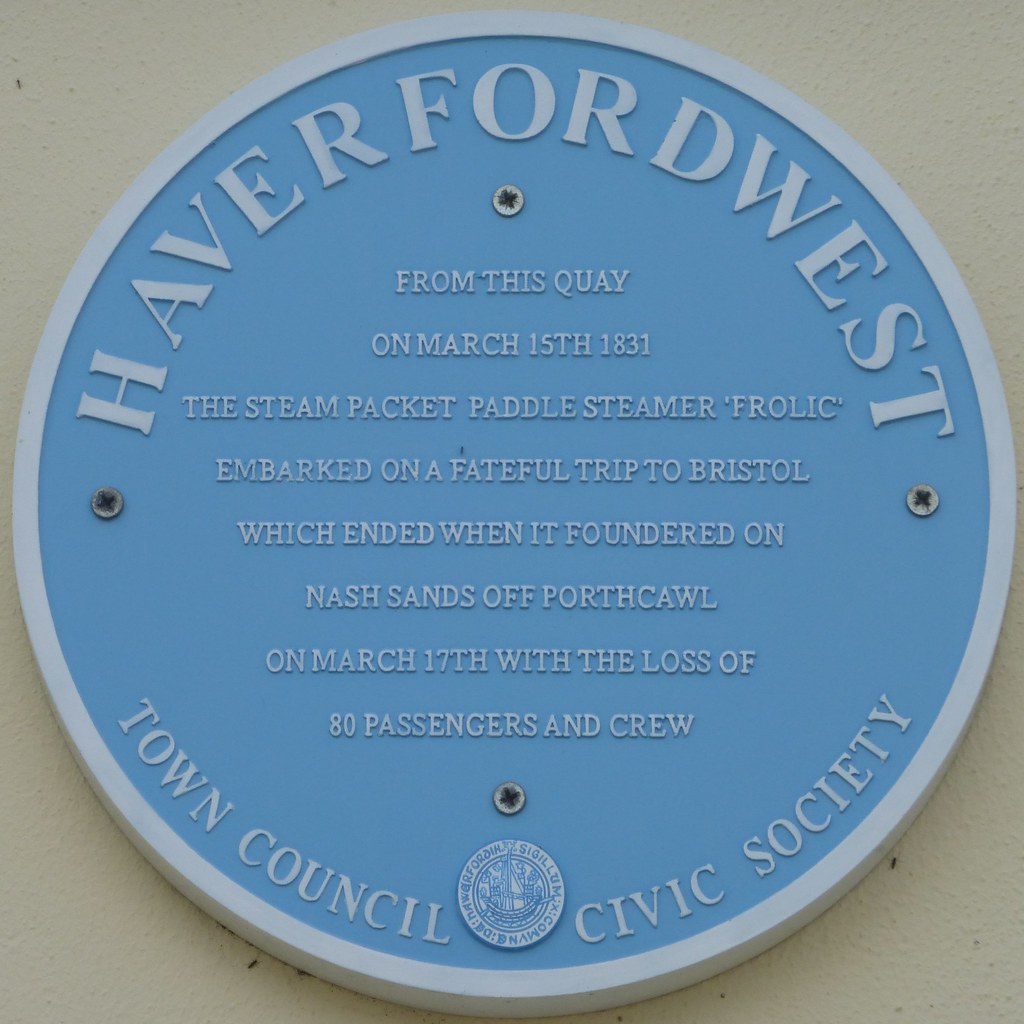This photograph features a round memorial plaque set against an off-white background. The plaque, prominently centered in the image, appears to be an outdoor installation in the middle of the day, likely near a historical site. The plaque itself is pale blue with a white border and contains raised white lettering that arches along the top, reading "Haverford West." The detailed inscription recounts a tragic maritime event: "From this quay on March 15th, 1831, the steam packet paddle steamer Frolic embarked on a fateful trip to Bristol, which ended when it foundered on Nash Sands off Porthcawl on March 17th with the loss of 80 passengers and crew." At the bottom, it states, "Town Council Civic Society," with a circular emblem situated between the words "Council" and "Civic." The plaque is affixed with four screws, one on each cardinal point. The colors visible in the image include shades of tan, white, light blue, silver, and gray.